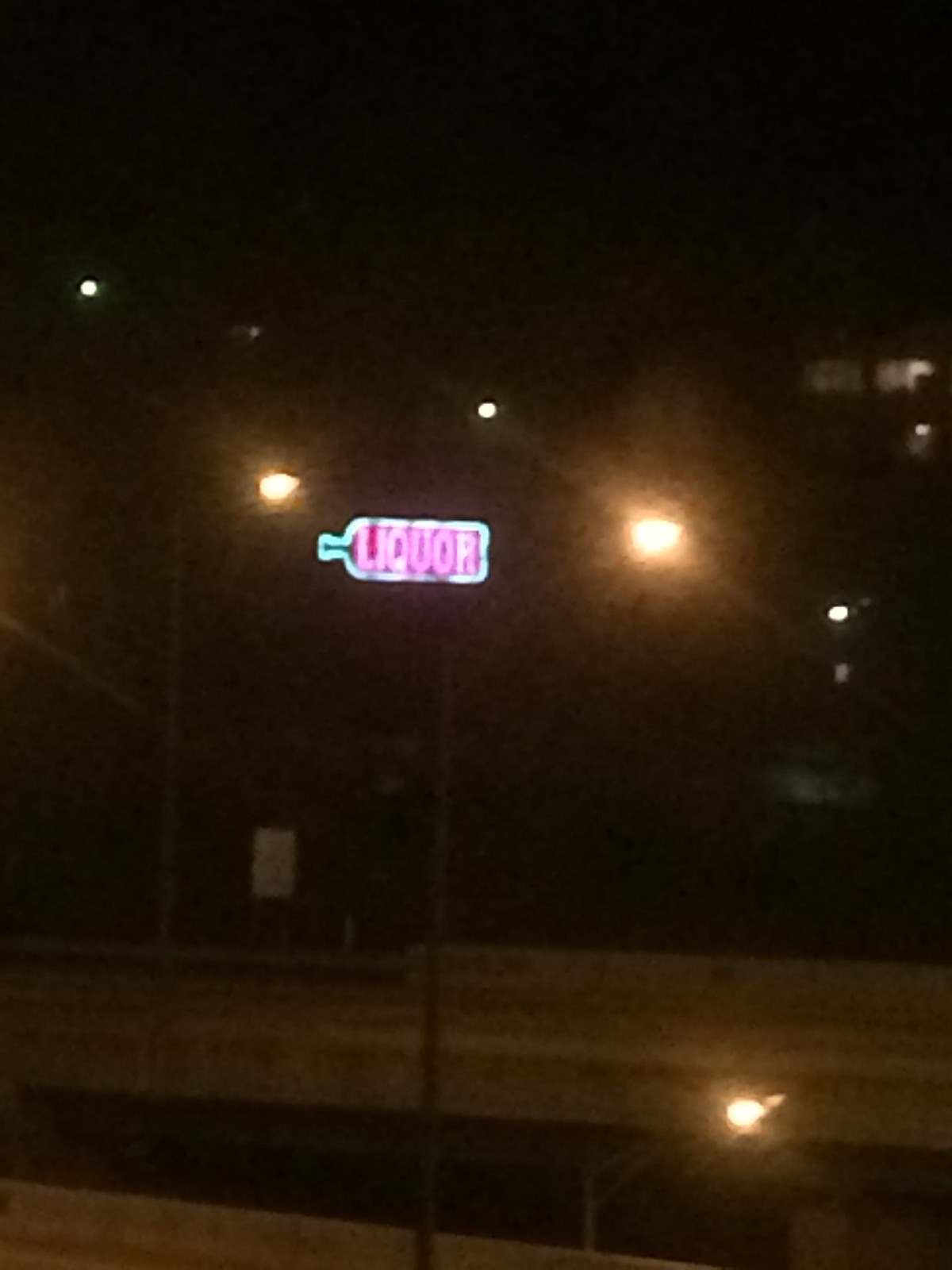This is a very low-resolution, blurred nighttime photograph of an outdoor city scene. The sky is completely black, providing a stark contrast to several small, white lights that are faintly visible on the horizon, possibly emanating from buildings or streetlights below. The far background suggests the presence of an apartment complex or house, partially illuminated by lights behind curtains.

Dominating the center of the image is a small, prominently glowing neon sign. The sign, shaped like a bottle laid on its side, features red fluorescent lettering spelling out "LIQUOR," which fills the entire bottle. Surrounding the red letters is a blue fluorescent outline of the bottle. To the left and right of this neon sign, two very bright and blooming lights cast a whitish-orange glow, likely from outdoor lamps attached to metal poles.

Below the neon sign, the image shows a light gray cement bridge or walkway. The walkway appears suspended, further adding to the layered complexity of this urban nightscape. Despite the blurriness, the vivid neon sign and subtle environmental details create a compellingly atmospheric scene.